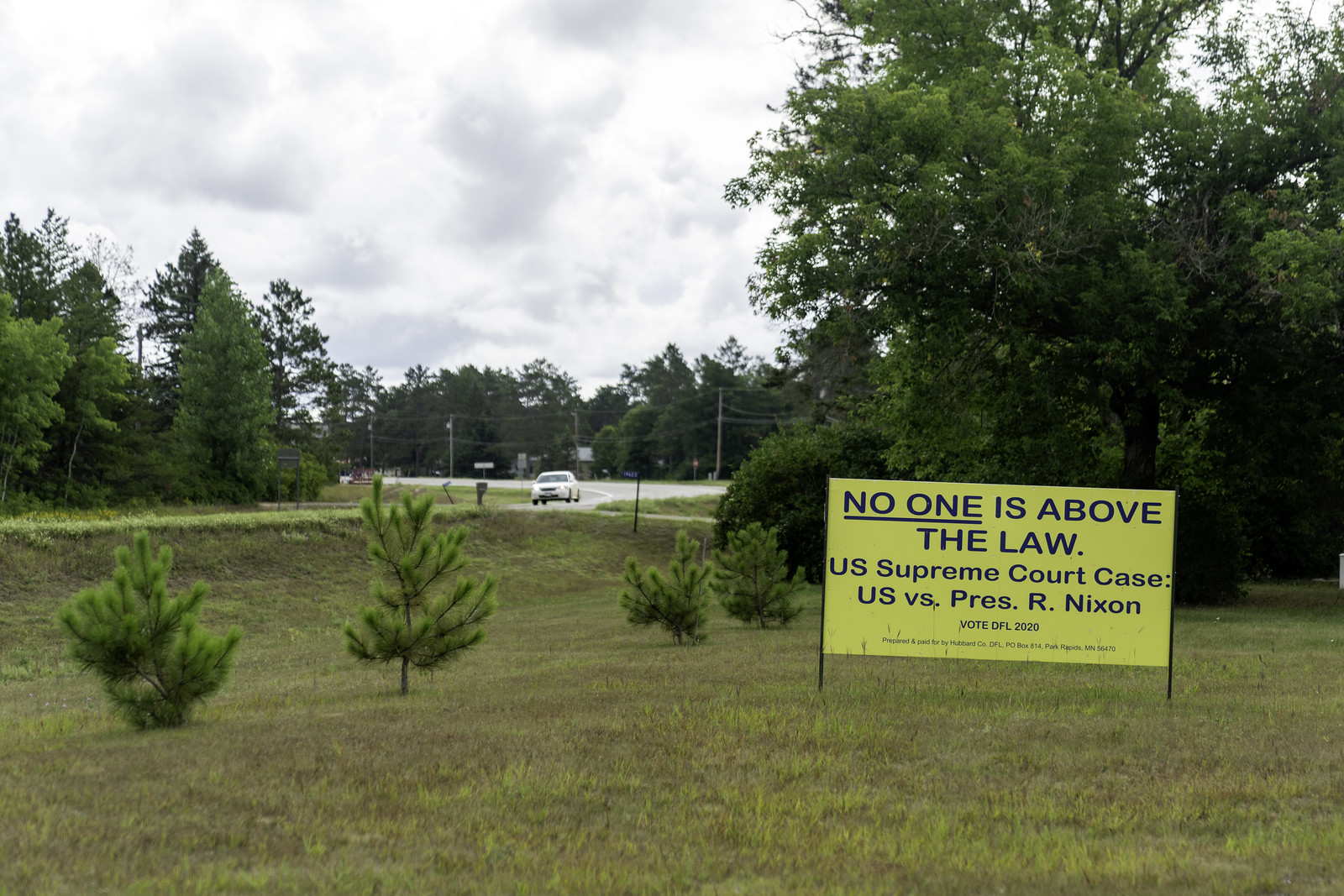A mostly cloudy sky with patches of blue stretches above a landscape dominated by trees. Tall trees frame the image from the left, right, and middle. In the foreground, a car is visible on the road. A yellow road sign on the bottom right reads "No one is above the law," referencing the U.S. Supreme Court case, United States v. Nixon. The ground beneath is a dry grass field. At the bottom left corner, there are several spiny fern leaves or branches diagonally spread out, significantly smaller compared to the taller trees that surround them.